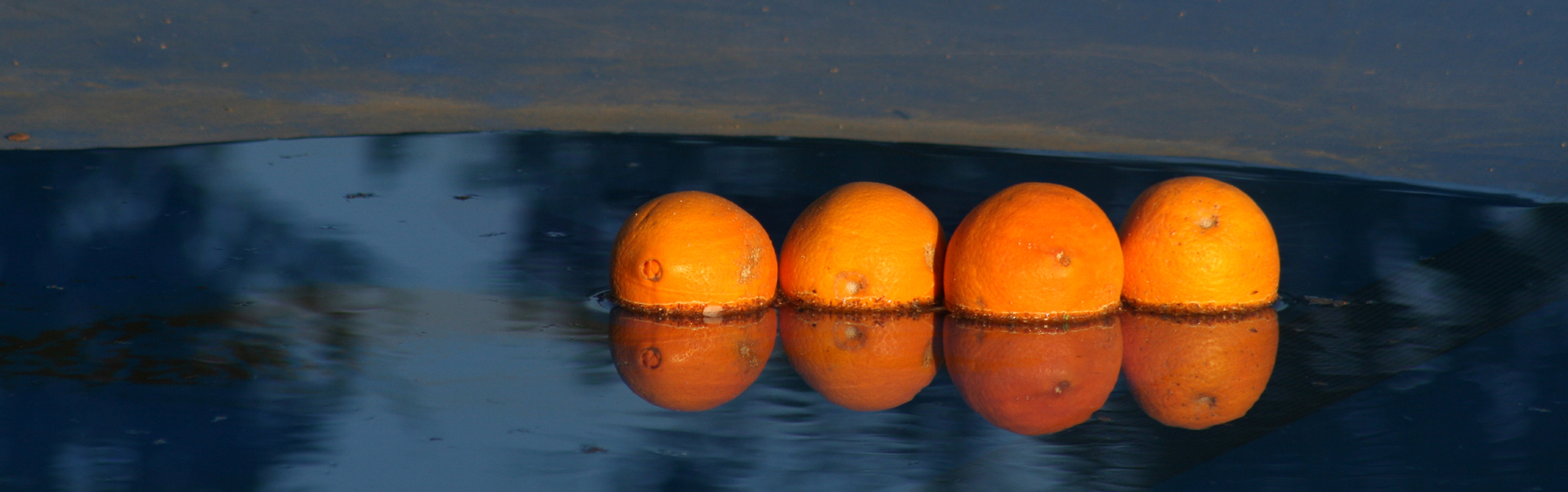The image presents a surreal, almost painting-like scene of four unblemished, round oranges seemingly floating in a pool of dark blue water. These oranges, aligned horizontally just off-center to the right, cast faint reflections on the water's surface, suggesting a close-up view. Above, the background transitions from a deep bluish-gray sky streaked with dark tan hues to an indistinguishable horizon, adding to the surreal quality. The water, marked by subtle ripples and slight color variations, mirrors the oranges but distorts their reflections, creating an otherworldly aesthetic. The overall impression is one of serene, uncanny stillness, with no text interrupting the composition.